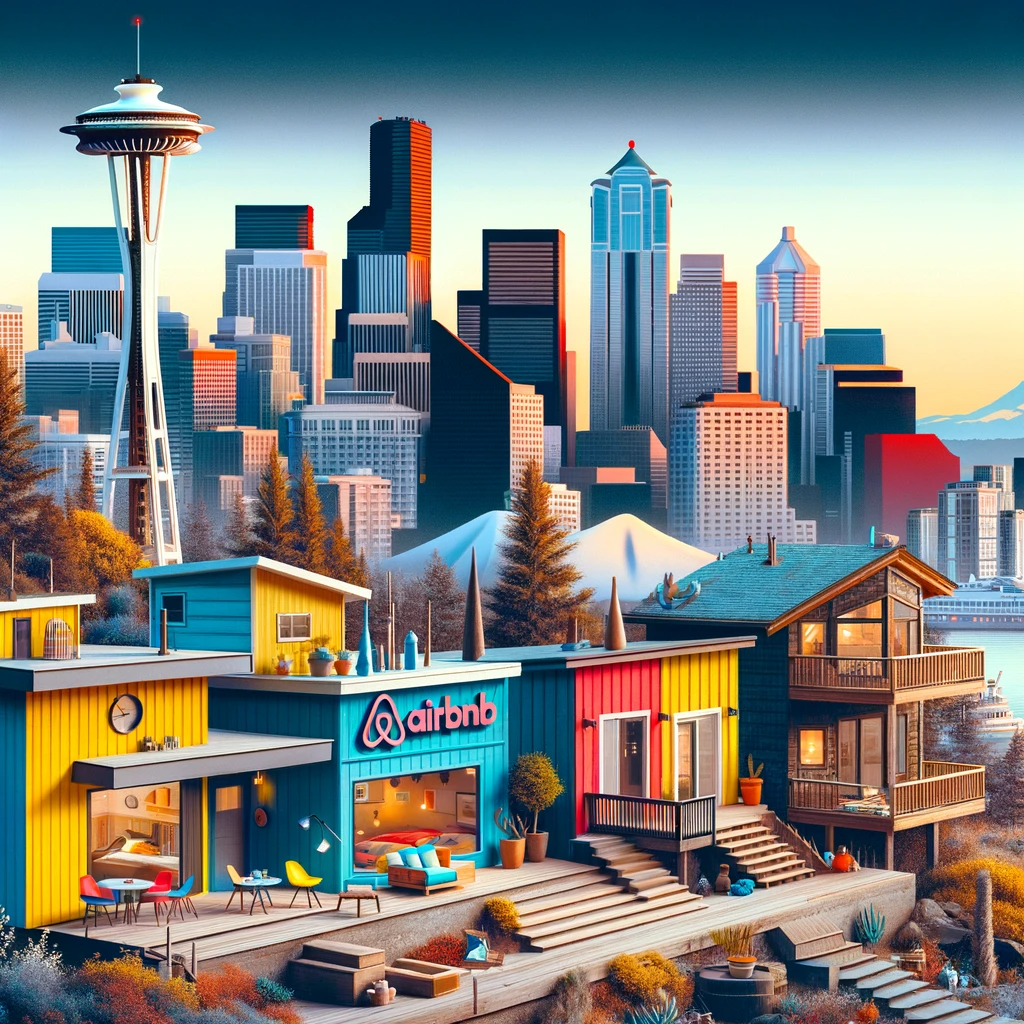This detailed, high-quality computer animation depicts the bustling Seattle skyline with its iconic Space Needle on the left, characterized by its hourglass design and UFO-like top with a red-tipped antenna. The cityscape features a mix of tall skyscrapers with bluish and reddish hues, hinting at reflections from the setting sun. Sizable buildings with numerous windows and horizontally striped façades extend into the background with shorter ones populating the foreground. Between these structures, trees in seasonal transition shades of brown and gold peek out. 

In the foreground, several colorful, wooden-style shacks add vibrancy with one prominently displaying the Airbnb logo against its blue panels, and an interior living area visible through a glass façade. This area includes multi-level decking adorned with bucket seats in yellow, red, and blue hues, surrounded by shrubs and plants. Stairs descend from the decking, partially trailing out of the bottom right corner. On the back right, a river flows with a few boats partially obscured, while the horizon transitions through a navy blue band to a lighter yellow behind the skyscrapers, subtly hinting at a mountain partially peeking from the right side.